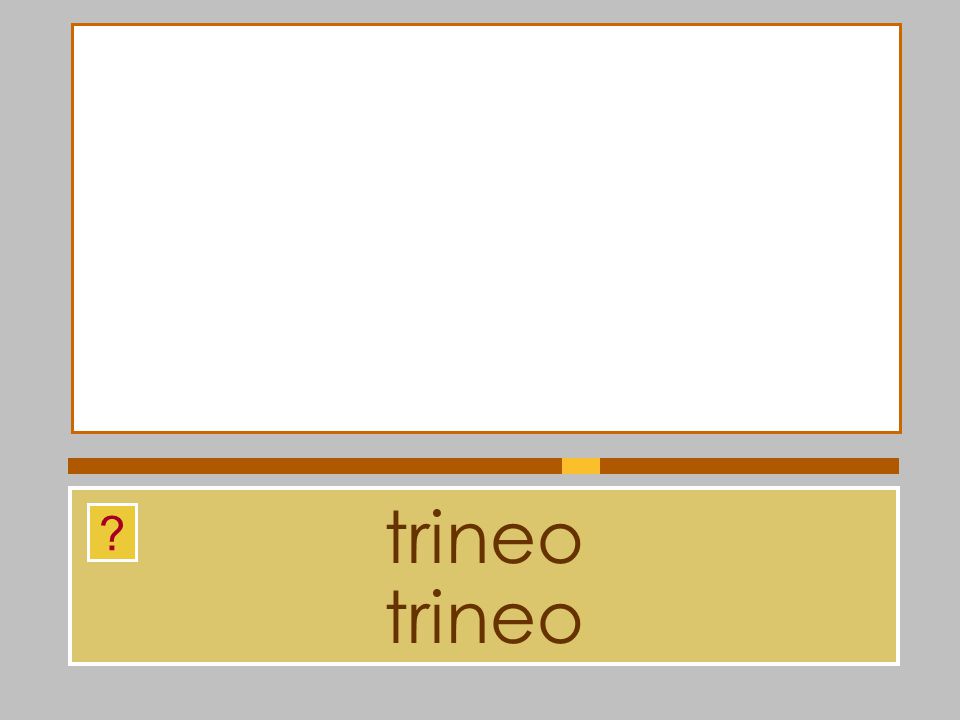In the center of a gray background, a large, empty, white rectangle is bordered by an orangish-brown frame. Beneath this is a thick dividing line in the same orangish-brown color featuring a yellow strip about 60% along its length. Below this line, a thinner rectangular box appears, bordered by a thin white line and filled with a tan color. To the upper left of this tan box, a small yellow box with a red question mark is situated. Centrally within this tan box, the word "Trineo" is repeated twice in dark brown, perfectly aligned text. The overall design feels incomplete, as if intended to be part of a larger, unfinished flashcard.